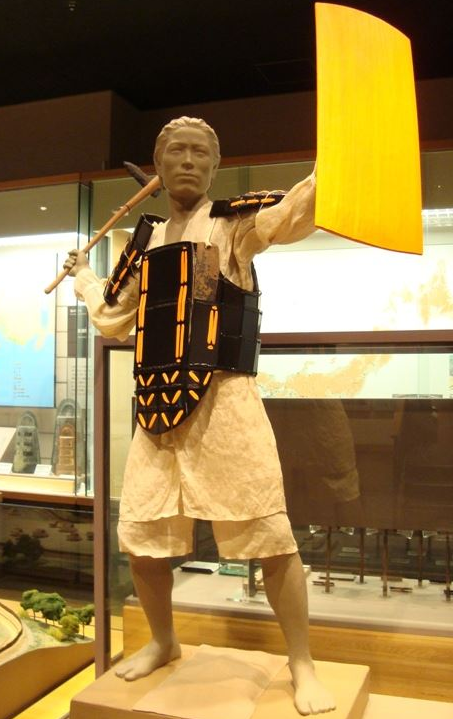This is a photograph of a life-size statue depicting a man, likely placed in a museum exhibit as inferred by the glass pane and wall with windows and lights in the background. The statue itself is made from a tan clay material and portrays a figure with a broad face, strong cheekbones, a strong chin, and short wavy hair that is not differentiated by texture from the rest of the sculpture. The man's outfit appears to be a combination of ancient and utilitarian attire. He is wearing a white linen garment, which could either be a shirt and shorts combination or a jumpsuit, along with a prominent black vest or armor that features yellow-orange striped accents protecting his chest and shoulders. His feet are bare, and his legs are exposed from the knees down.

In his left hand, the man is holding a gold or yellowish wooden rectangular shield, while his right hand, cocked back as if prepared to strike, grips a wooden stick with a sharp black triangular stone or metal piece at the end, reminiscent of an ice pick or hatchet. The statue stands on a low pedestal, enhancing its exhibition-like presentation. The predominant colors in the scene are various shades of tan, white, orange, and black, adding to the historic and rustic aesthetic.